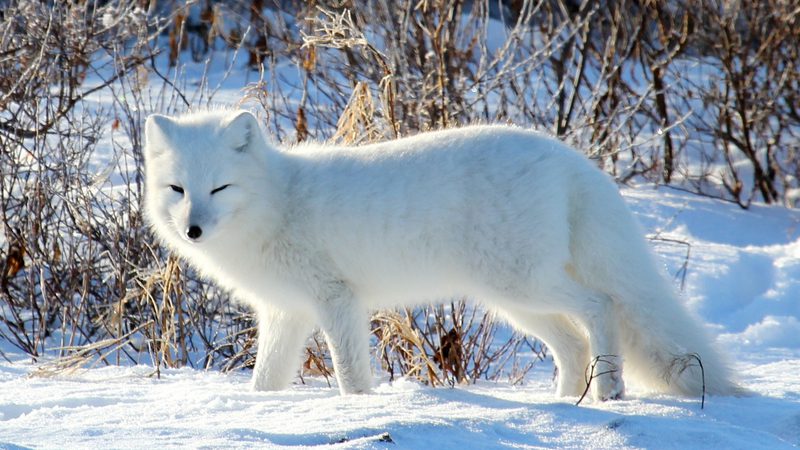This is an image of a white arctic fox standing out in the snow, captured in mid-walk. The fox is centrally positioned, with its big, bushy white tail to the right and its head, featuring small black eyes and a little black nose, to the left. The fox's fur is very thick and fluffy, which is typical for a cold-weather species. Its eyes are almost closed, giving the impression that it is squinting. The snowy ground is about ankle-high to the fox, and behind it, there are leafless trees, dead brown branches, and grass poking out of the snow, adding a stark contrast to the pristine white environment. The fox seems to be moving towards some sunlight, and its gaze is directed at the camera, making for a striking and cool image.